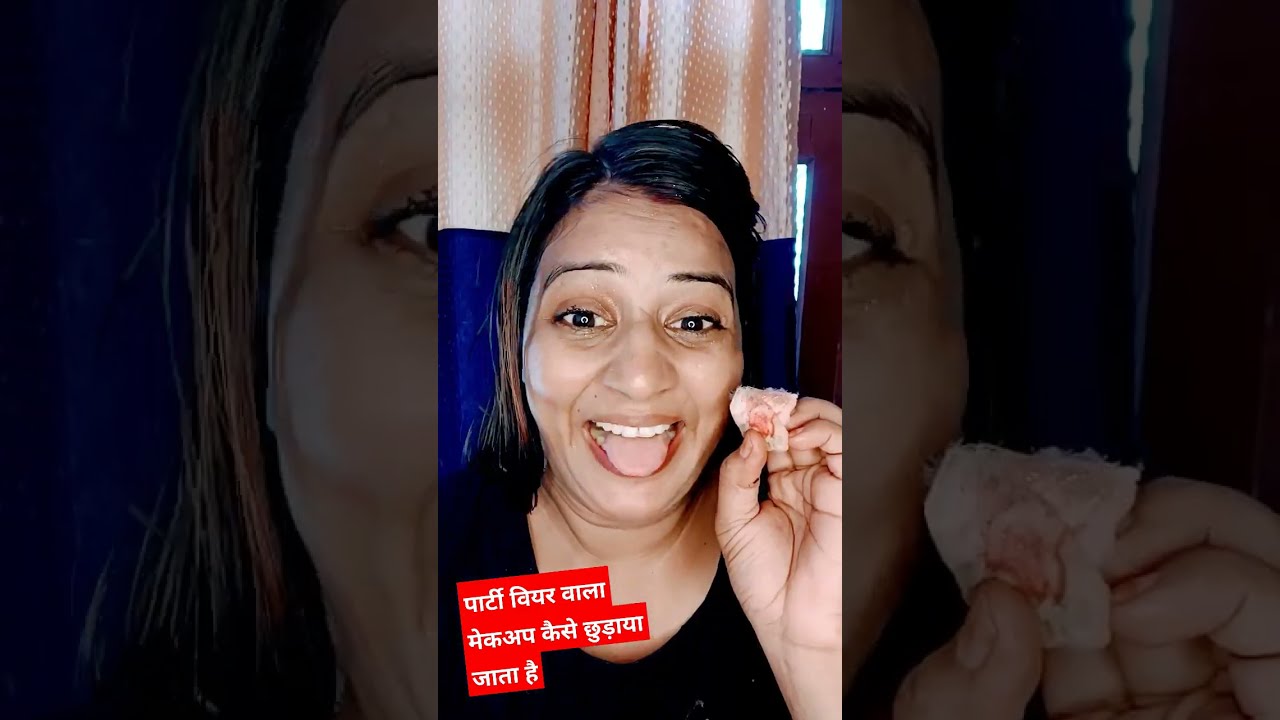The image depicts a woman, likely of Southeast Asian descent, with caramel-colored skin, dark eyes, and dark greasy hair that is black with a hint of brown on one side. She is wearing a black top and appears to be very excited, indicated by her open mouth with a protruding tongue and a big grin that reveals her very white teeth. The woman is holding an item in her left hand, possibly a light pink piece of food or a material with an image, though its exact nature is unclear. In the foreground, there is a red caption box with white text at the bottom left corner, likely in a foreign language, possibly Hindi or Arabic.

The background features a blue chair and a curtain that is light pink at the top and blue at the bottom, with holes in the upper section. Behind the curtain, there are windows framed in maroon or red, suggesting it is daytime outside. The image has a border on both sides, which is a grayed-out close-up of the woman's face and hands from the central portion of the image, creating a repeating effect.